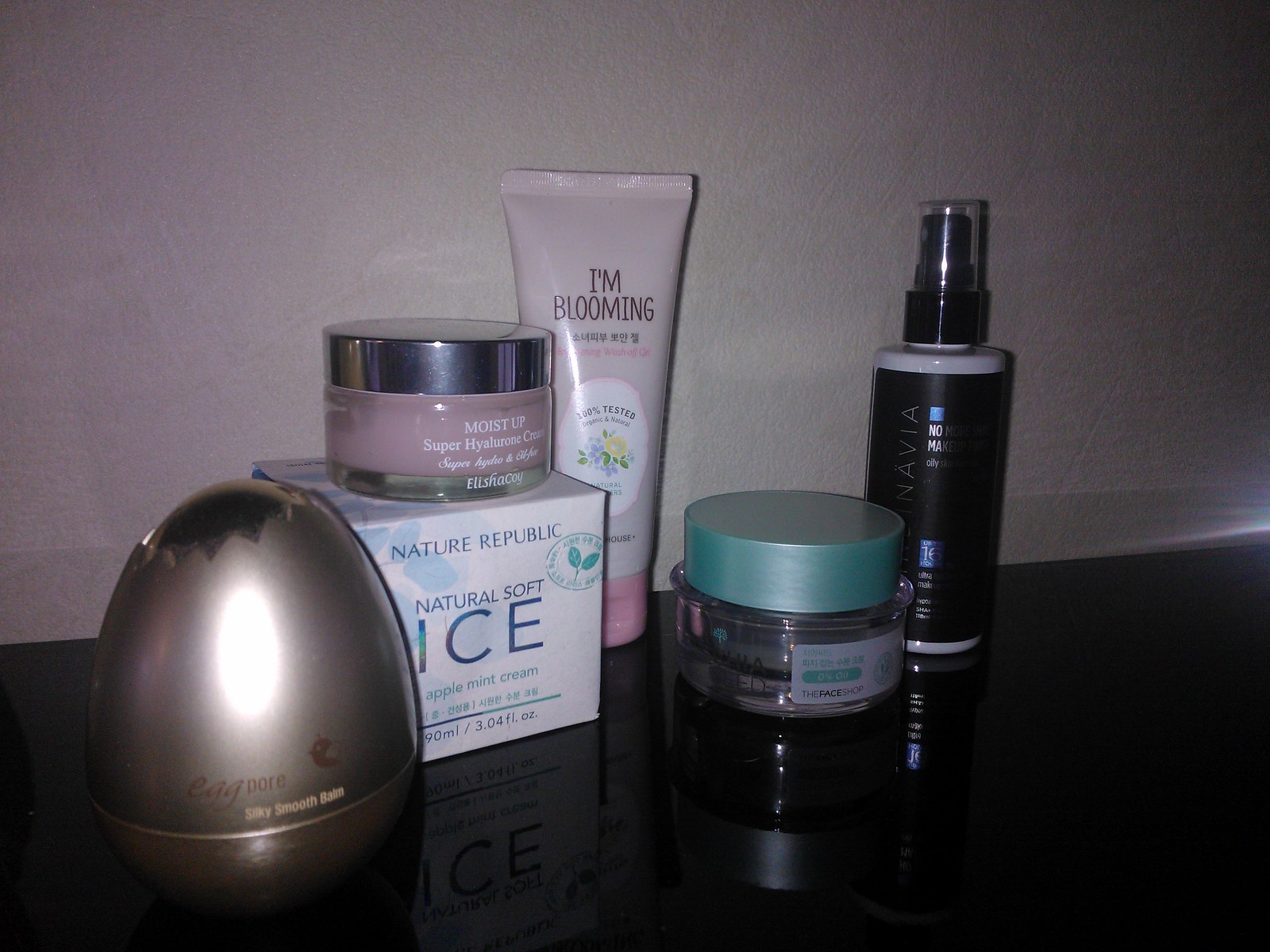The image showcases a collection of beauty products meticulously arranged on a sleek, black, shiny laminate table, positioned against a minimally decorated wall, likely adorned with plain white or greyish wallpaper. The table holds six distinct items, each contributing to a well-curated aesthetic.

1. **Egg Pour Silky Smooth Balm**: This item stands out with its unique egg shape and golden-brown color, embodying both elegance and charm.
2. **Nature Republic Natural Soft Ice**: Immediately to the right, this 3.04 fluid ounce apple mint cream is encased in a pristine white box, exuding a sense of purity and freshness.
3. **Moist Up Super Hyaluron Cream**: Positioned atop the Nature Republic box, this glass tub with a striking silver lid contains a visually appealing pink product, promising hydration and vitality.
4. **I'm Blooming Cream**: This eye-catching pink tube with floral decorations features predominantly Chinese writing and notable phrases such as "100% tested." The darker pink lid rests at the bottom, grounding the product in an upright position.
5. **Unidentified Clear Liquid in a Green-Lidded Glass Tub**: This small, translucent container with a green plastic lid holds a clear liquid. Despite the small, illegible writing, its compact design hints at a potent formulation.
6. **Navia Black Spray Bottle**: The final item in the lineup, this sleek black bottle with a transparent cap on the sprayer maintains an air of mystery due to its barely discernible label, suggesting a refined, modern product.

The arrangement on the glossy surface, coupled with the neutral backdrop, amplifies the clean and sophisticated appeal of the beauty essentials on display.